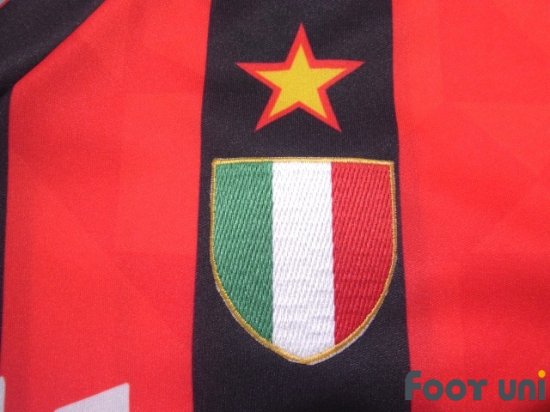This is a very close-up photograph of a section of red fabric, likely from a uniform or jersey. Prominently displayed on a black stripe running down the fabric is a gold star rimmed in red, situated above what appears to be the red, white, and green stripes of the Mexican flag. The backdrop itself is a deep red, and the material hints at being a piece of cloth or fabric. In the bottom right-hand corner, the text "Foot Uni" is inscribed in black, with the dot on the 'i' uniquely colored yellow. Interestingly, the top left corner of the image shows a small triangle of black, suggesting the fabric changes color at that point. Meanwhile, the bottom left corner reveals a small slanted triangle of white, possibly the tip of another design element on the fabric. This detailed section of the uniform suggests it might be related to football, in the soccer sense, hinting at a player's jersey.